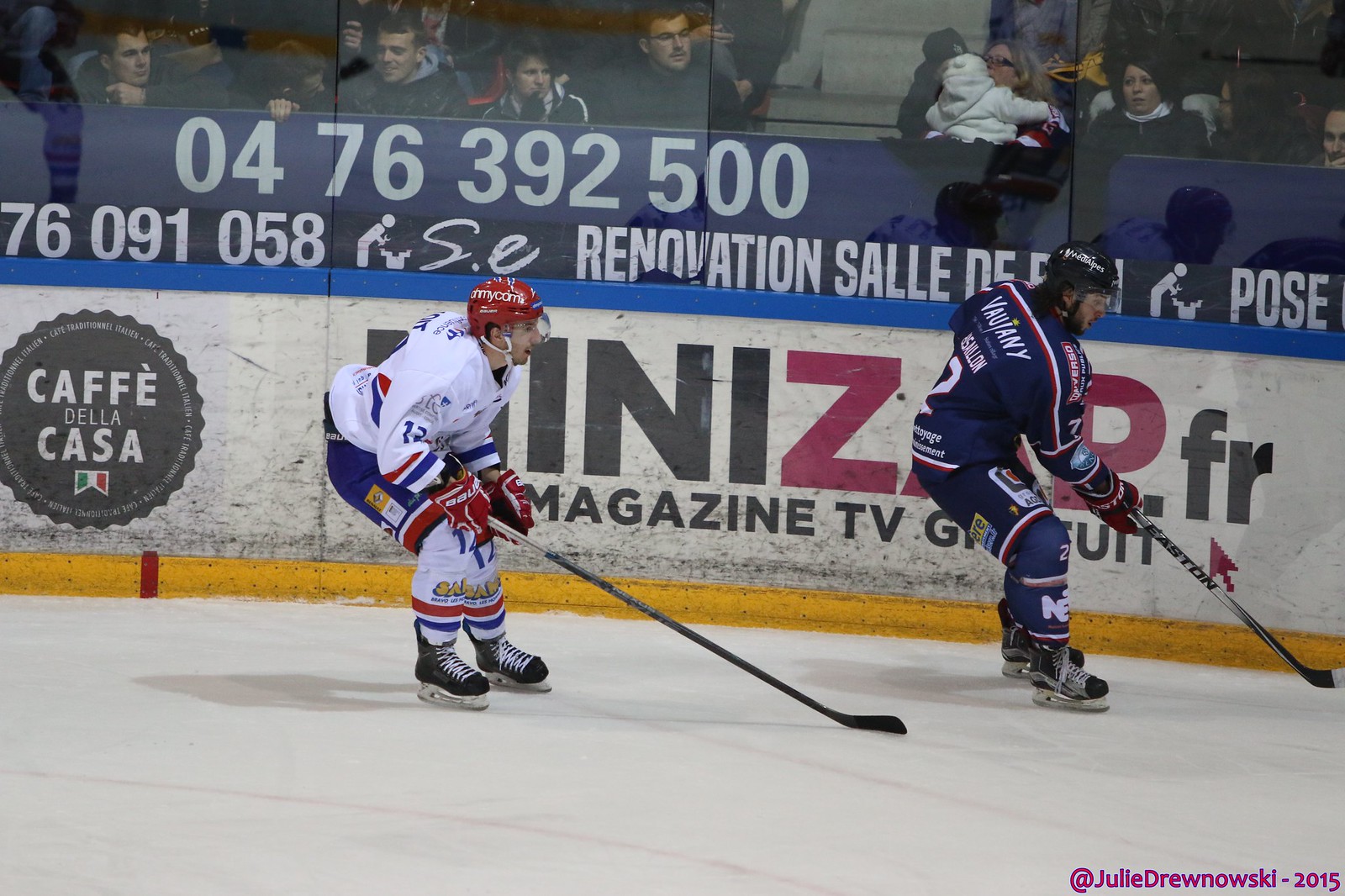The image captures an intense moment during an ice hockey game, showcasing two players in action on the rink. The player in the foreground is dressed in a predominantly white uniform with blue shorts and a red helmet, gripping a hockey stick as they advance towards the puck. Close by, another player from the opposing team is clad in a navy uniform with red stripes and a black helmet, also holding a hockey stick and seemingly in pursuit of the puck. Behind the players, the audience watches from the stands, partially obscured, with their faces not clearly visible. The wall along the rink is adorned with advertisements, including a partially visible sign with the phone number "0476392500" and an ad for "Cafe Casa." The rink's perimeter is white, featuring steps and additional signs in various languages, enhancing the competitive atmosphere of the game.